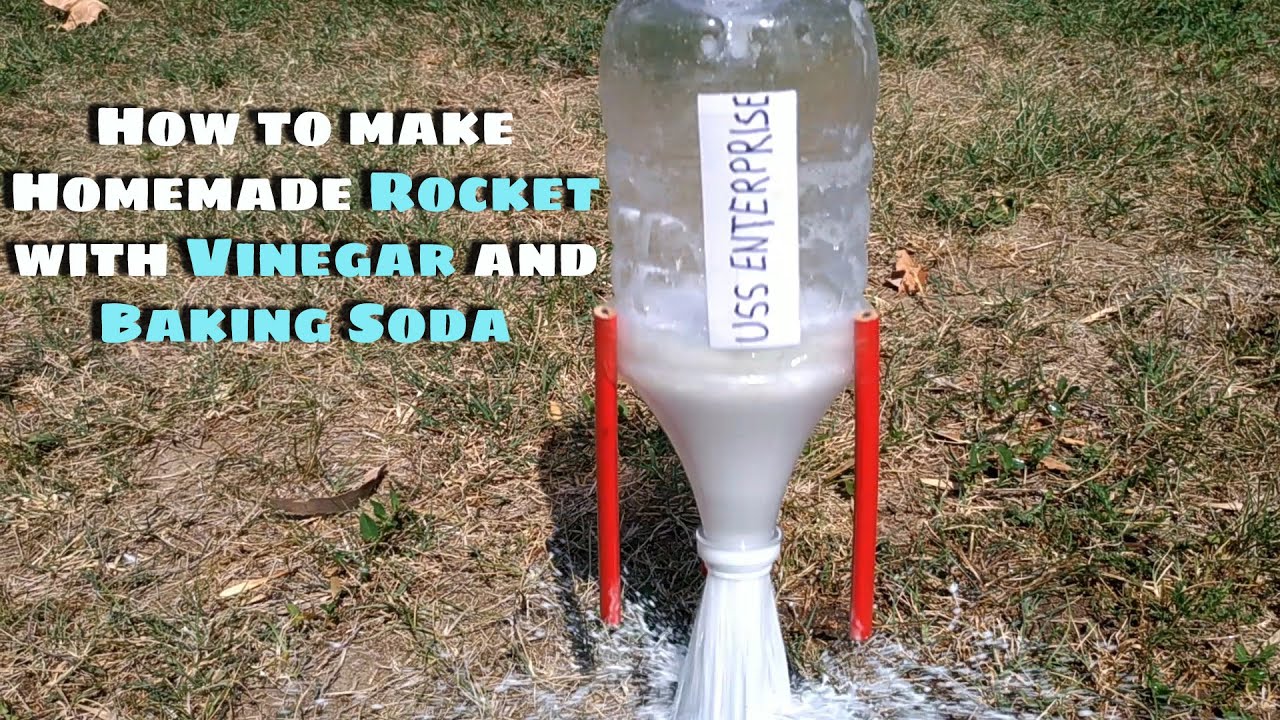The image is an eye-catching advertising banner for a guide on creating a homemade rocket using vinegar and baking soda, likely meant for educational purposes such as a YouTube thumbnail. Positioned in the top left corner, the banner features four lines of text: "How to Make" in white, "Homemade" in white and "Rocket" in blue, "with" in white, "Vinegar" in blue, and "and" in white, followed by "Baking Soda" in blue. 

The photograph prominently displays a two-liter plastic bottle upside down, partially filled with a white solution, spilling out from the neck to simulate propulsion. The bottle appears to be rocketing off a grassy field, aided by this stream of white liquid. Attached to the bottle are two red pencils, one on each side, functioning as makeshift stabilizers.

Adding a personalized touch, the bottle is labeled with a white tag that reads "USS Enterprise" in black handwriting. The scene is set against a green and brown patch of grass, enhancing the outdoor experimental vibe.

In summary, the detailed banner image visually combines educational content with a playful, practical demonstration of a homemade rocket, creating an engaging and informative visual guide.